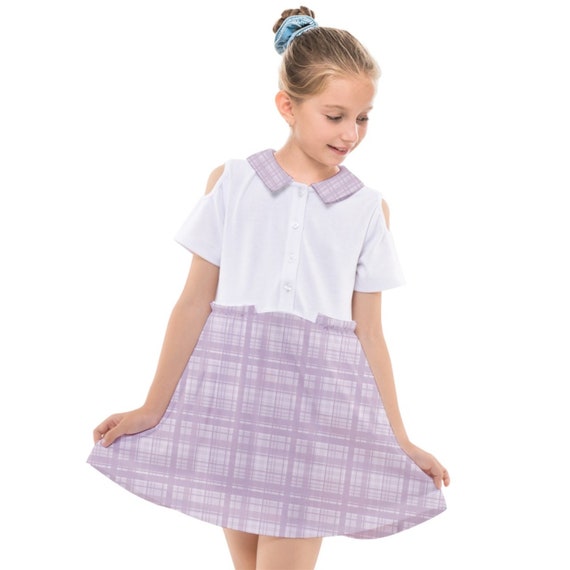In the image, a young Caucasian girl, likely around 10 years old, is standing against a completely white background, giving the impression that her outline has been superimposed onto it. She showcases a charming and playful pose, holding out the sides of her dress as if performing a curtsy, reminiscent of Mary Poppins or a classic model pose. Her hair, blonde and neatly styled, is pulled back into a bun secured with a thick, baby blue scrunchie. She glances downward and to her right with a gentle smile.

The dress she's modeling is a one-piece garment that could be pulled over the head. The top part is white and features a purple plaid collar resembling a lumberjack's checked shirt, coordinating with the bottom of the dress, which shares the same pinkish-purple plaid pattern. The dress exposes her bare shoulders and forearms, contributing to a summery and casual look. The detailed plaid design and the harmonious blend of colors and patterns suggest that this image might be intended for an online advertisement or a magazine spread, depicting the girl in a fashionably light and poised manner.